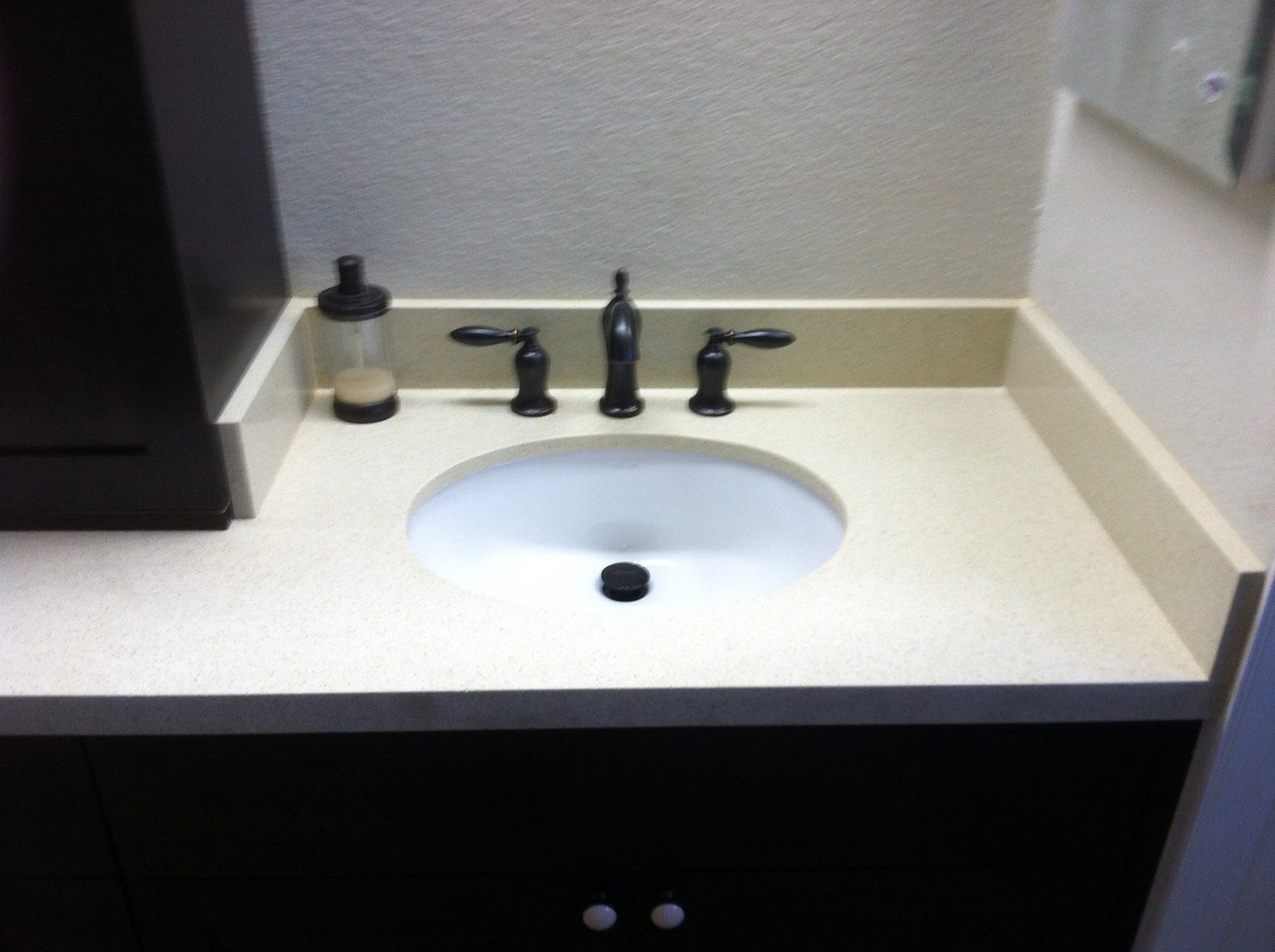In this bathroom sink area, the sink itself features a pristine white base complemented by black handles and a matching black sink stopper. The white countertop and back wall create a clean, cohesive look. On the left, there is a sleek black soap dispenser filled with a brown liquid, adding a touch of contrast. To the right of the sink, a mirror is mounted on the wall, reflecting the tidy space. Below, a drawer with two white handles offers additional storage. A prominent black pillar on the left side frames the scene, enhancing the modern aesthetic.